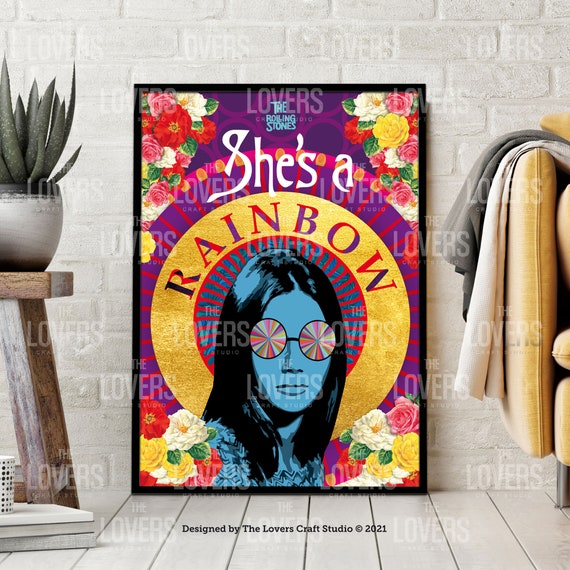This is a promotional poster for The Rolling Stones, featuring a striking artistic representation. At the very top of the image, the word "Lovers" is prominently displayed in purple lettering. Directly beneath this, the band's name, "The Rolling Stones," is written in bold blue text.

The centerpiece of the poster is an eye-catching image of a woman painted in vivid blue tones. She sports a pair of multi-colored glasses resembling pinwheels, adding a dynamic element to her appearance. Her black hair, tinged with blue highlights, complements her blue attire, which merges seamlessly with her blue complexion.

Adding to the psychedelic aesthetic, the phrase "She's a Rainbow" is written in white text against a vibrant purple and red background adorned with flowers at all four corners.

To the right side of the poster, a wooden table in a brown hue is visible, topped with a green plant housed in a white vase. Further to the right, set against a white wall and floor, there is a gold-colored chair with a blanket draped over its arm, enhancing the overall scene's texture and depth. This detailed amalgamation of elements suggests the poster's purpose as a promotional artwork for The Rolling Stones, reflecting their iconic and flamboyant style.